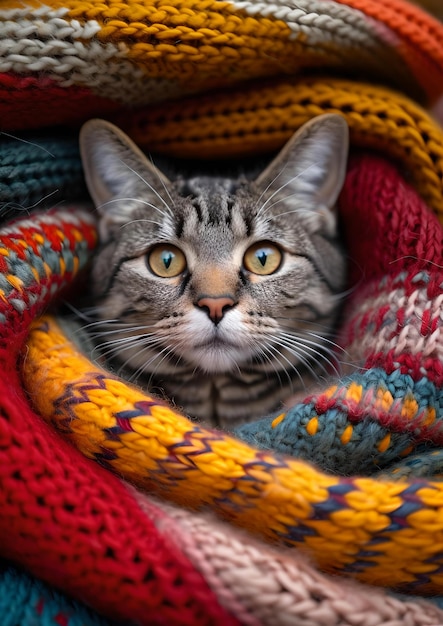This is a detailed photograph featuring a gray and black striped tabby cat, wrapped snugly in a multi-colored knit scarf. The cat's fur is predominantly gray with black stripes, with a touch of brown above the nose and white inside the ears. Its big, bright eyes—generally described as either green or yellow—are wide open, conveying an extremely surprised expression. The cat's ears are erect, and it stares directly at the camera, making for an engaging and somewhat comical portrait. The cat is surrounded and swaddled by a large, cozy scarf that blends a variety of warm, fall colors, including orange, red, green, white, and blue, making it look very warm and comfortable. The scarf's vibrant hues and patterns, potentially knitted or crocheted, add a rich texture to the image, enhancing the cozy and colorful setting that frames the cat's startled yet endearing face.